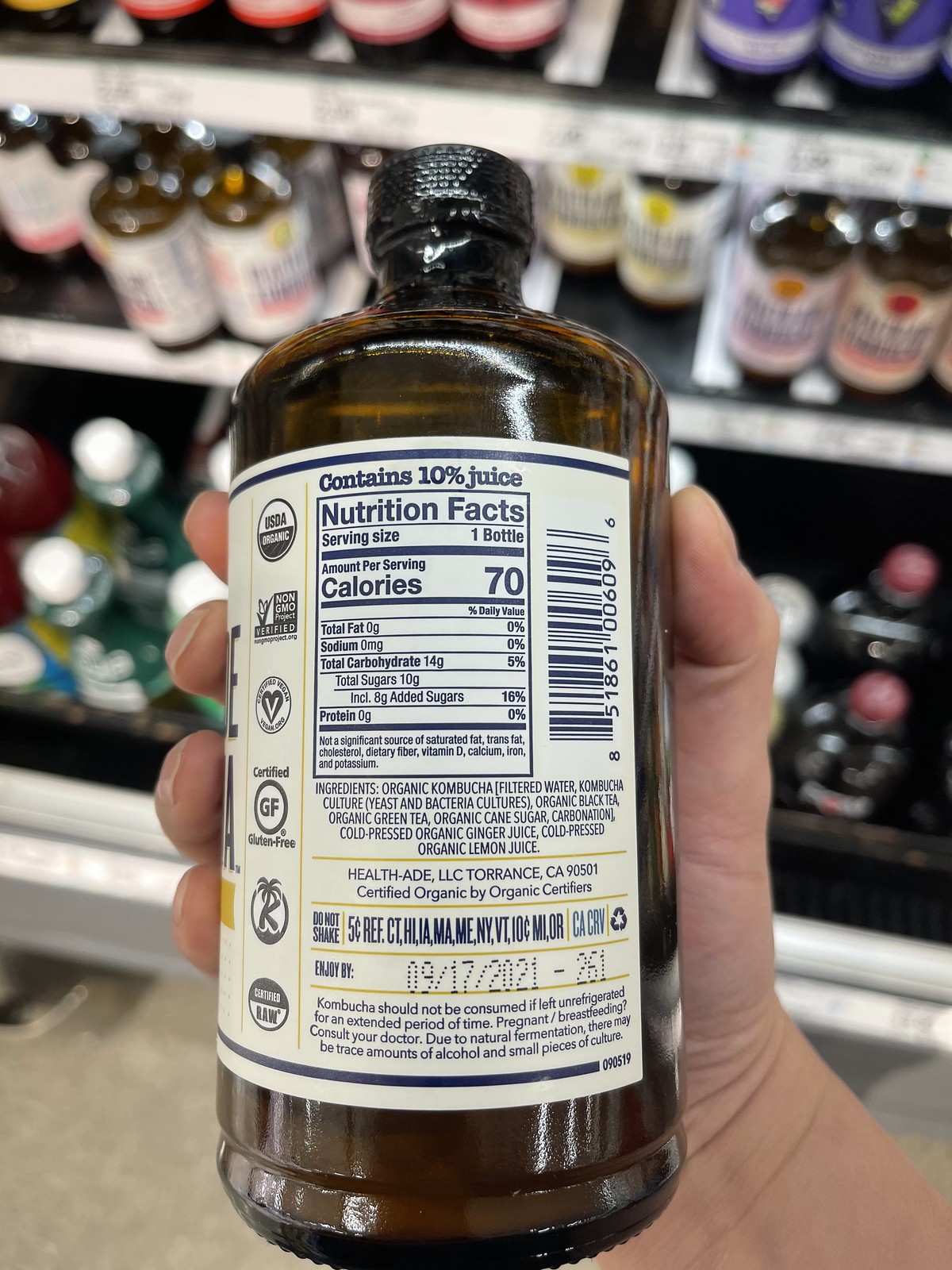In this detailed photograph, a man is holding a cylindrical, amber-colored bottle with a short neck and a black cap up to the camera, prominently displaying its nutritional facts label. The label, printed on white with several yellow lines, provides key information such as USDA organic, non-GMO certified, gluten-free, kosher, certified raw, 70 calories, 10% juice, and ingredients, including details about trans fats, sodium, carbohydrates, and protein. The bottle’s greenish-brown glass has multiple labels, including a barcode on the right-hand side. The setting appears to be a supermarket, evidenced by numerous similar bottles lined up on store shelves in the background. The man's hand, originating from the lower right corner of the photo, grips the bottle with four fingers on the left and his thumb on the right, emphasizing the beverage's detailed labeling and emphasizing its health-conscious credentials.